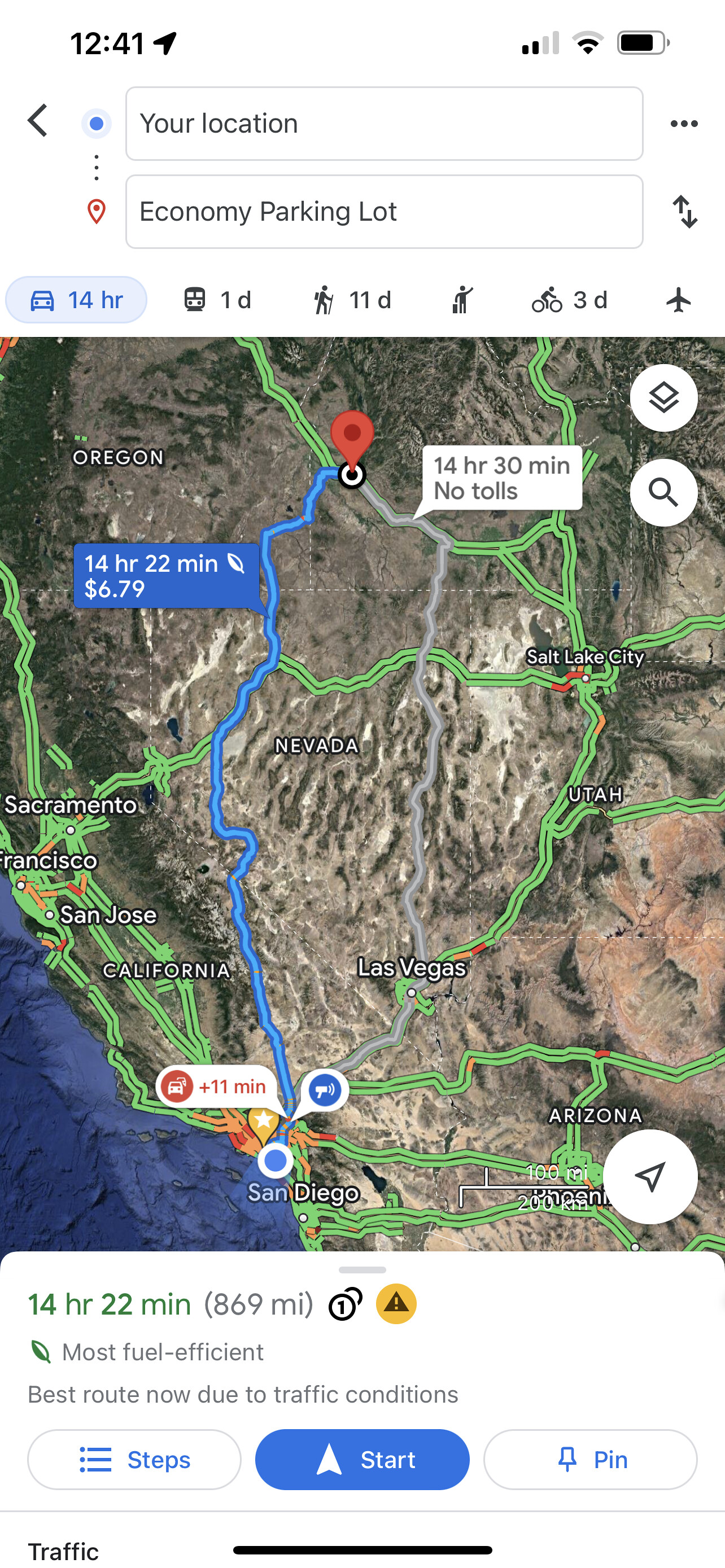This map displays a detailed route from San Diego, California, to a location in Idaho, potentially Boise, though the destination is not definitively identified. The map indicates a driving duration of 14 hours and 22 minutes, with a noted cost of $6.79, which likely represents an estimated expense, possibly related to electric vehicle charging. The map is somewhat disorganized and lacks the typical flat layout, but it highlights the most direct and fuel-efficient route. Green lines and bars illustrate alternative highway systems that, while less fuel-efficient, offer different travel options. Additionally, travel times for other modes of transportation are provided: one day by train, 11 days on foot, and three days by bicycle.